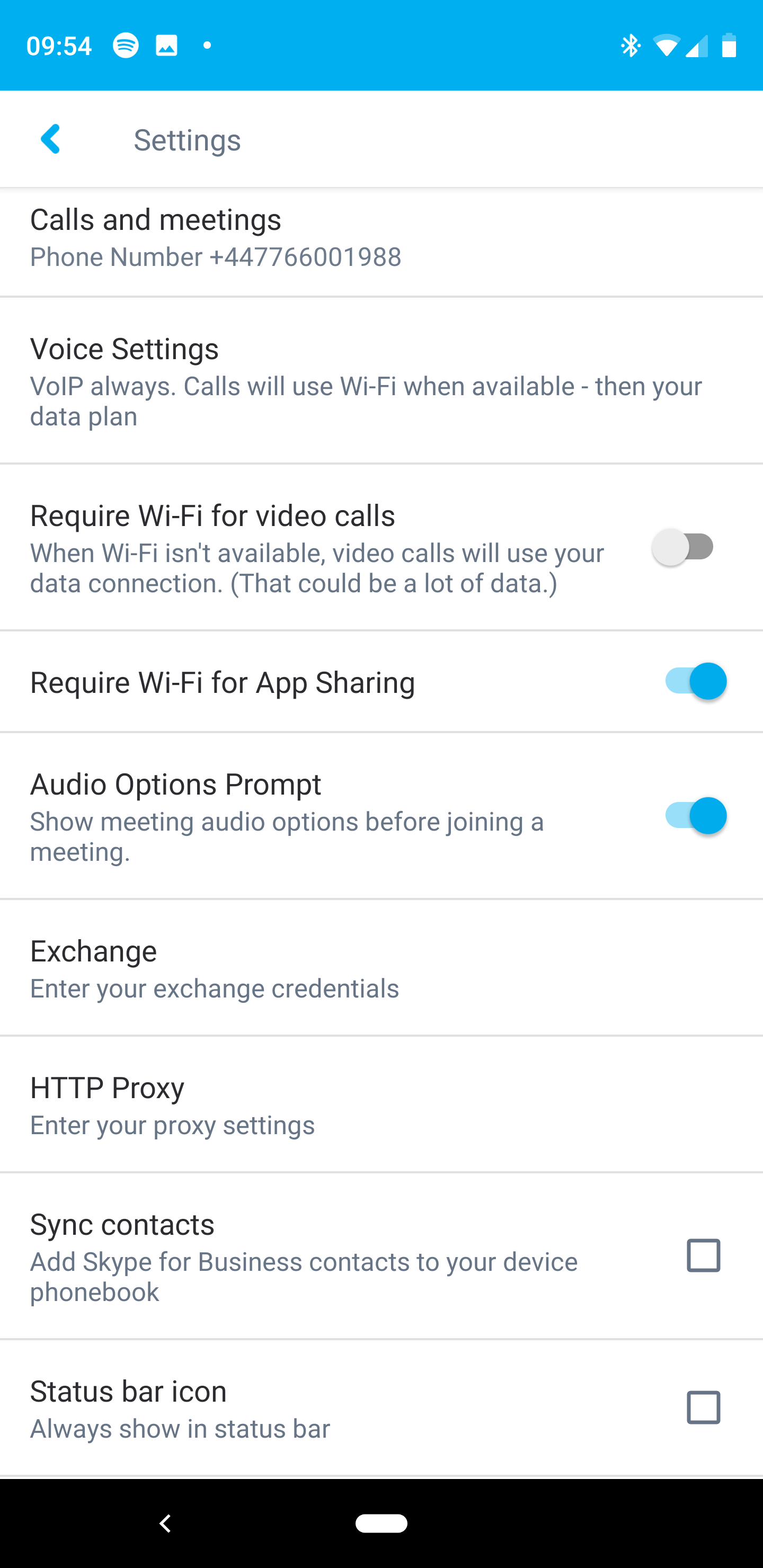**Detailed Caption:**

The image appears to be a screenshot taken from a smartphone. The top portion of the screen, often referred to as the status bar, features a blue background. On the top left, the time is displayed as "09:50," and to the right, there are several icons visible. These include a Spotify icon, a screenshot icon, a Bluetooth icon, a Wi-Fi icon, a network icon, and a battery icon. All of these icons are white.

The main content of the screenshot shows a settings page with a white background. The word "Settings" is prominently displayed at the top, followed by a list of settings options written in black text. The settings listed are as follows:

1. **Call Settings:** Displays the phone number "+44 7766 001988."
2. **Voice Settings:** Indicates the option "VoIP always call with," which will use Wi-Fi when available, followed by the data plan.
3. **Require Wi-Fi for Video Calls:** Notes that when Wi-Fi isn't available, video calls will use the data connection. This setting has a toggle switch, which is currently set to "off."
4. **Require Wi-Fi for App Sharing:** This setting is toggled on and the switch is blue.
5. **Audio Option Prompt:** Shows the option "Show meeting audio options before joining a meeting," which is toggled on.
6. **Exchange Credentials:** This option includes the ability to enter exchange credentials.
7. **HTTP Proxy:** Allows entering proxy settings.
8. **Sync Contact:** Features the setting "Sync Skype for Business contacts to your device phone book," which has a checkbox that is not checked.
9. **Status Bar Icon:** Displays the option "Always show status bar," which also has a checkbox that is not checked.

The detailed list is structured neatly, making each option easily distinguishable for the user.